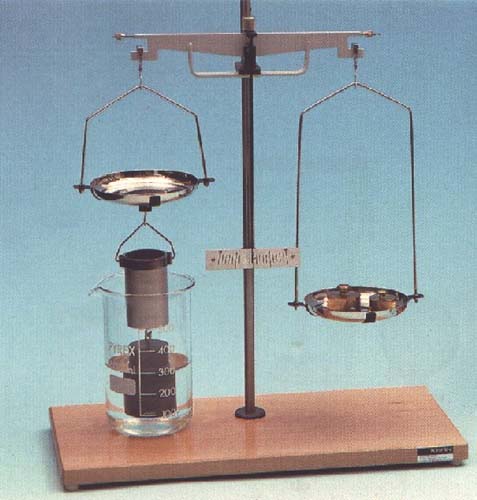The image depicts a vintage mechanical scale, prominently featuring a substantial rectangular wooden base set against an evocative gradient background that transitions from a lighter blue at the bottom to a darker blue towards the top. At the center of the wooden base stands a vertical metal rod anchored by a washer to protect the wood, providing stability and durability. At the top of this rod, a horizontal metal beam extends outwards. 

From either end of this beam, delicate hooks extend down to support two circular metal trays meant for weighing items. The right tray contains several thick metal discs, presumably acting as weights to measure objects against. The left tray, contrastingly, is empty of weights but instead suspends a cylindrical canister, roughly the size of a D battery, capped in black. This canister is housed within a transparent glass beaker marked with measurement lines, suggesting a scientific or laboratory context.

The detailed construction and setup of the scale, the presence of the beaker with measuring scales, and the use of metal weights all point towards a meticulous purpose, possibly for precise measurements in scientific experiments or lab work.